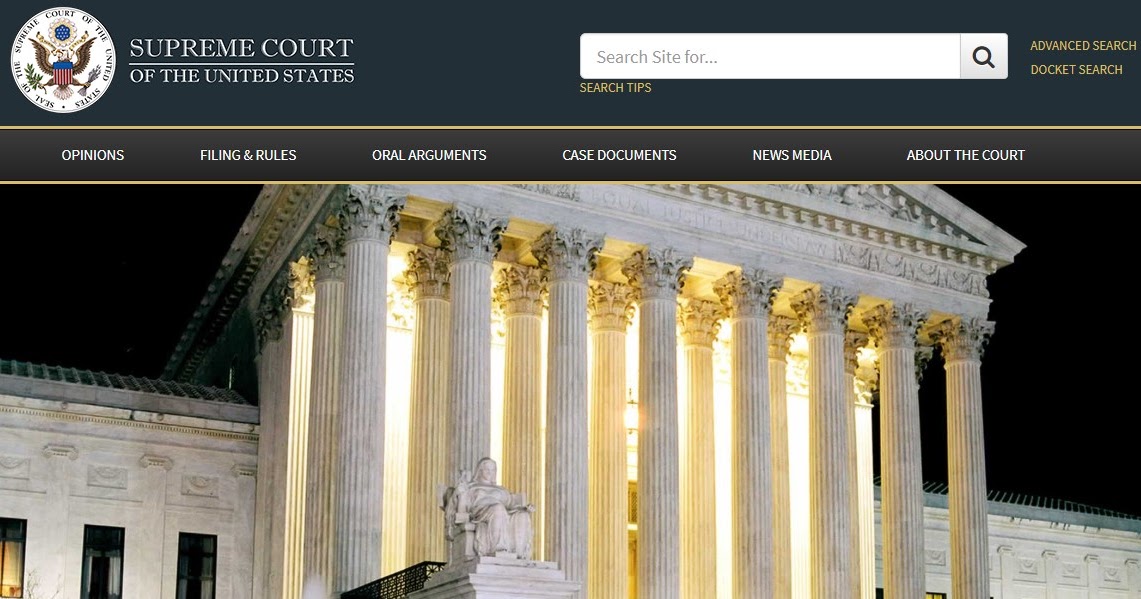The screenshot captures the homepage of the Supreme Court of the United States' official website. At the top of the page, a black banner stretches across, prominently featuring the official seal of the Supreme Court. This seal is a white circle containing a detailed eagle grasping ribbons and olive leaves in its claws, accompanied by the inscription, "Seal of the Supreme Court of the United States." To the right of the seal, the title "Supreme Court of the United States" is displayed in bold.

Beneath the banner, a white search bar invites users with the placeholder text, "Search site for... ," and is accompanied by a magnifying glass icon. Below this search field, a clickable link labeled "Search tips" offers guidance on how to effectively utilize the search function. To the right of the search bar, options for "Advanced search" and "Docket search" are available.

The website’s navigation is organized into six primary tabs: Opinions, Filing and Rules, Oral Arguments, Case Documents, News Media, and About the Court. Each tab directs users to specific information pertaining to various functions and resources of the Supreme Court.

Dominating the lower portion of the page is a striking image of the Supreme Court building at night. Illuminated by strategic lighting, the building's classical columns and a front-placed statue are bathed in a glowing light, highlighting the architectural grandeur and solemn atmosphere of the highest court in the United States.